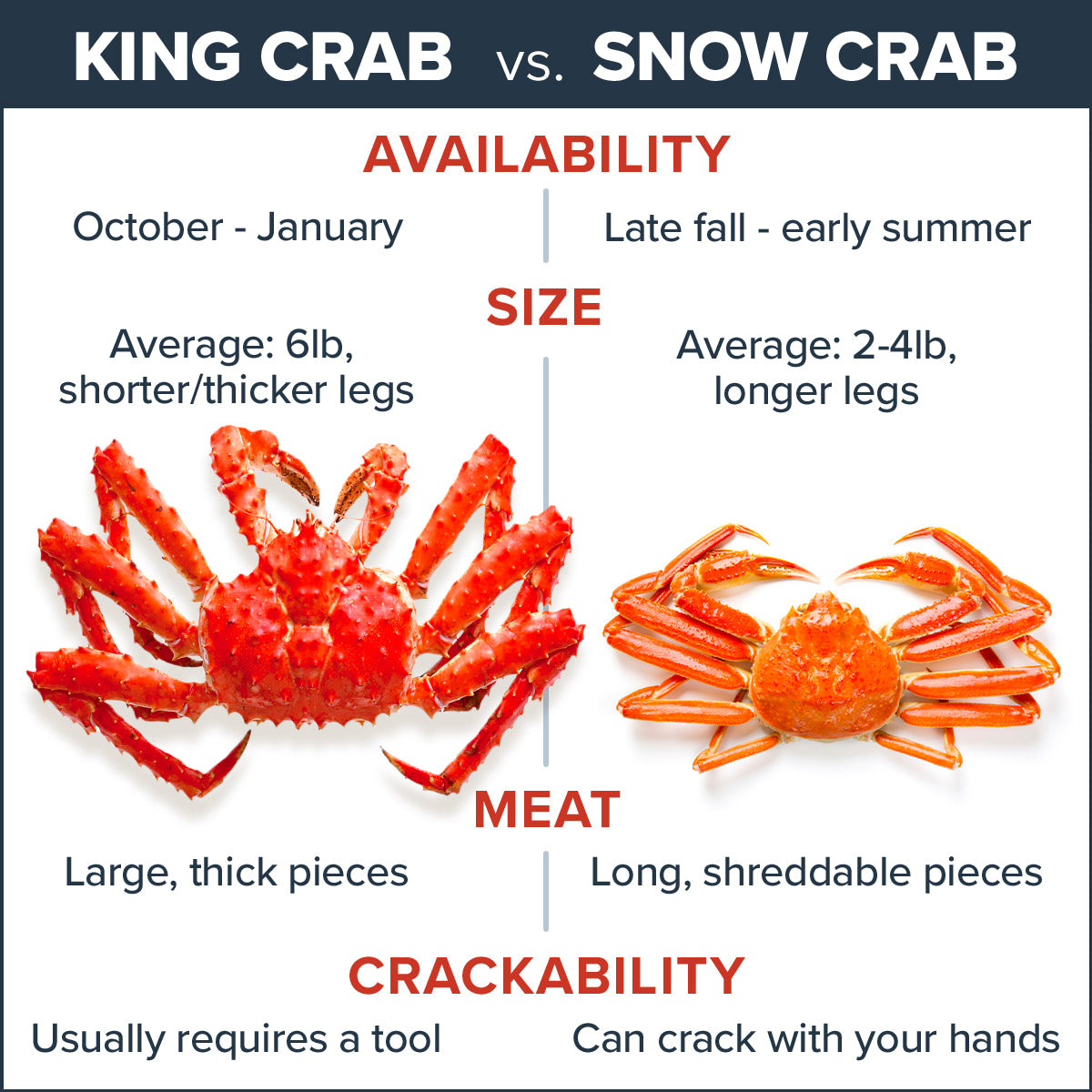This poster provides a detailed comparison between King Crab and Snow Crab. At the top, the title "King Crab vs. Snow Crab" is prominently displayed. The comparison includes various categories: 

- **Availability:** King Crab is available from October to January, while Snow Crab is available from late fall to early summer.

- **Size:** The King Crab averages 6 lbs and has shorter, thicker legs, whereas the Snow Crab averages between 2 to 4 lbs with longer legs.

- **Appearance:** The picture shows the King Crab on the left, which is larger and red in color, whereas the Snow Crab on the right is smaller, with a more orange hue and longer legs.

- **Meat:** The King Crab offers large, thick pieces, while the Snow Crab has long, shreddable pieces.

- **Crackability:** King Crab meat usually requires a tool to crack, whereas Snow Crab can be cracked open with your hands.

The background of the image is white, and the text is mostly in blue and red, providing a clear and colorful contrast to the crabs' illustrations.